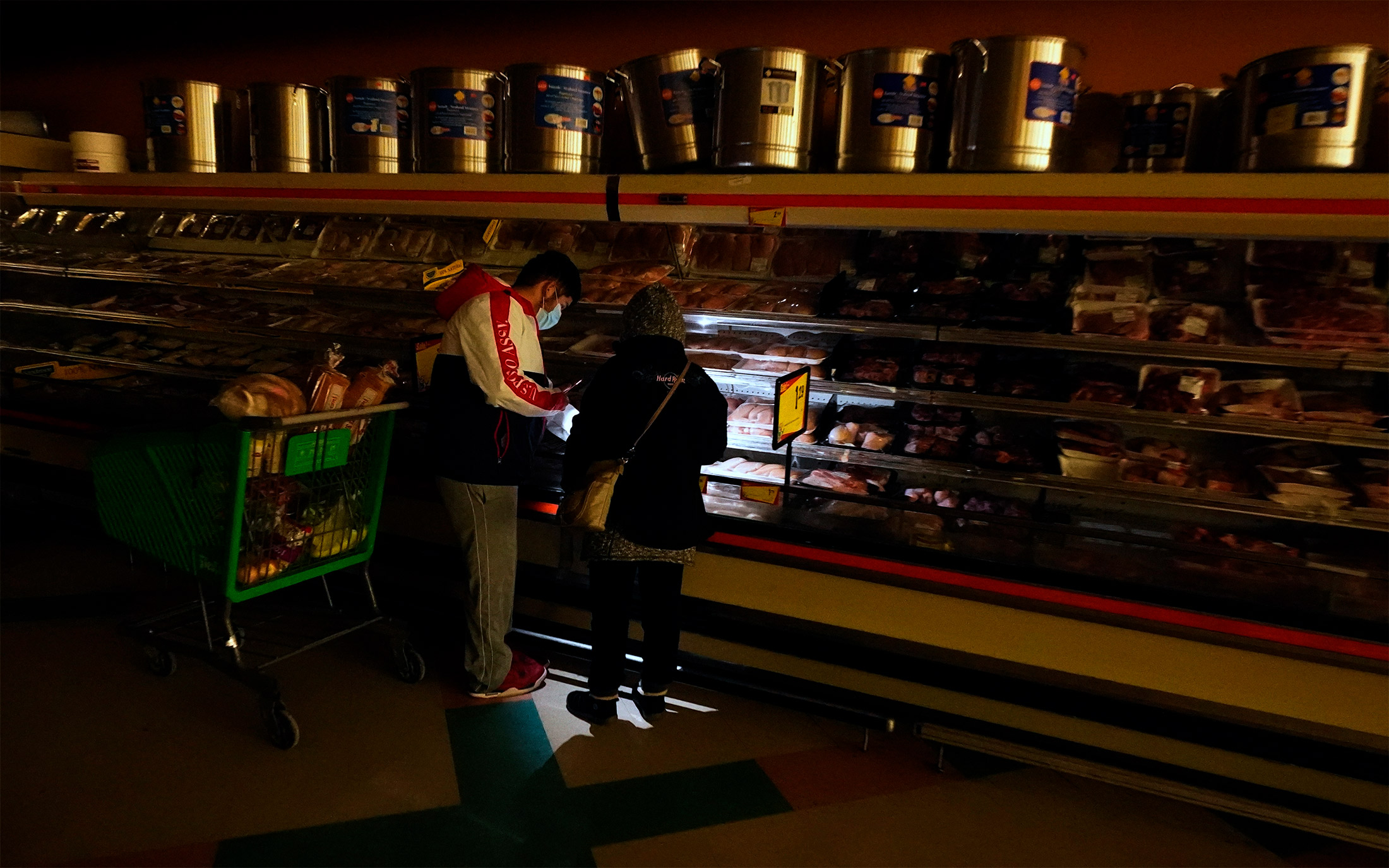In this dimly lit image of a grocery store, the power appears to be out, casting the meat section in shadows. Customers rely on flashlights to navigate the dark aisles. In the foreground, a man in a white and red jacket, blue medical mask, and gray pants focuses his flashlight on the packaged meats, each labeled with its name and price. Beside him, a woman with a yellow purse, black jacket, and black pants examines the selection. A green shopping cart filled with groceries, including a loaf of bread, stands nearby. Above the refrigerated meat cases, a row of large, shiny stainless steel pots, reminiscent of those used for cooking turkey or making gumbo, lines the top. The cooler features a white top border with a red stripe running along its length, adding a touch of color to the otherwise dark scene. A yellow sale sign highlights a special offer among the neatly packaged meats.